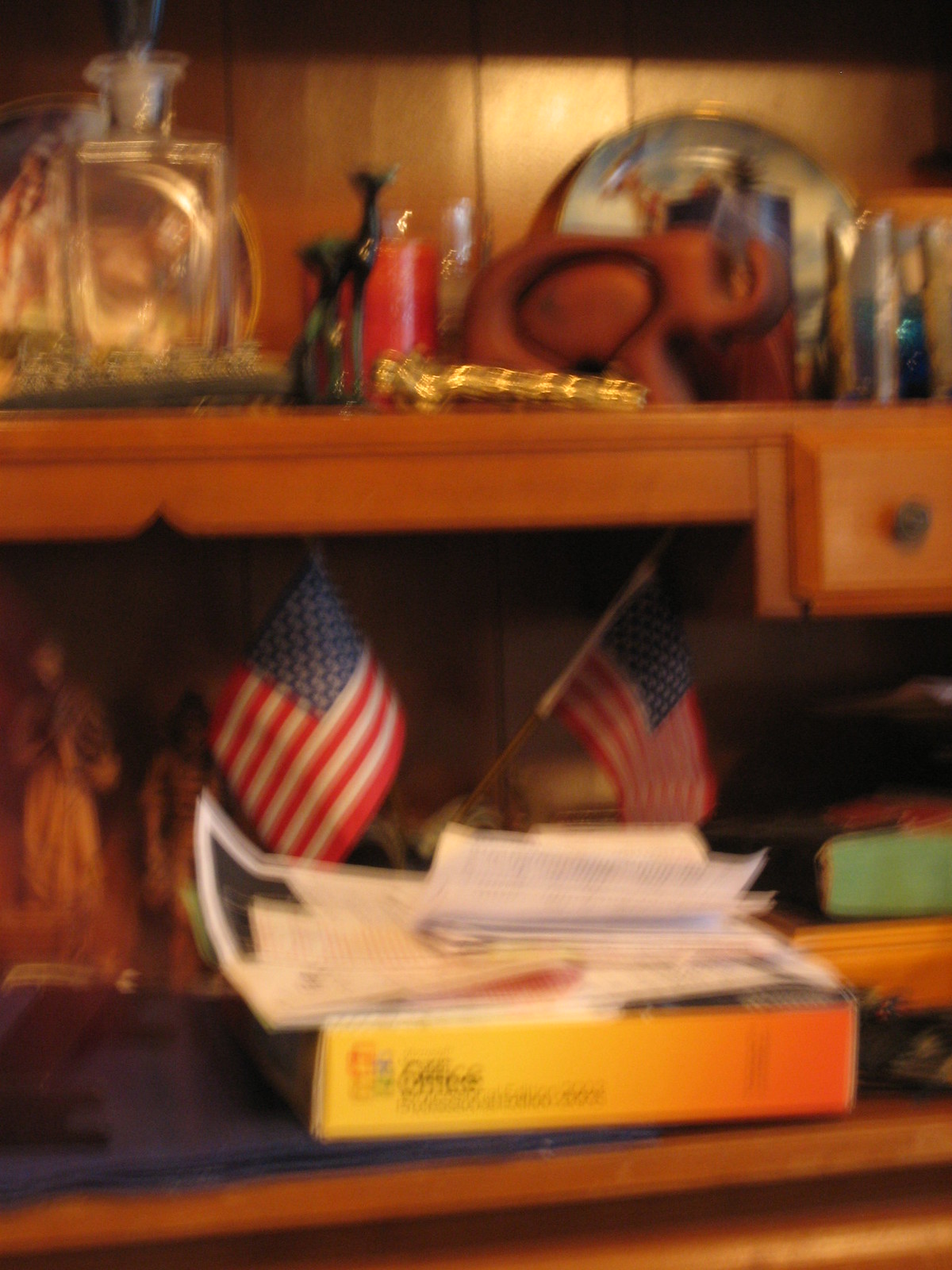This image depicts a slightly blurred office desk adorned with various items. Central to the image, on the bottom shelf of the wooden desk, is a yellow-to-orange, sunburst-colored Microsoft Office box with "office" clearly readable. This box is flanked by two American flags positioned in opposite directions. Above the box, a series of colorful papers, likely some folded flyers and documents, are layered. To the right of these flags is a ceramic figurine, and to the left, a light blue book is visible.

The desk's top shelf features an assortment of trinkets and knickknacks. On the far left, partially visible, is a wooden drawer knob. Next to it stands a photo or cologne bottle, surrounded by a collection of small perfume bottles and a gold item. A notable decorative plate, a wooden elephant, a glass bottle, which might be a snow globe, and possibly the back of a clock also occupy the shelf. The backdrop includes a wood-inspired color palette, complemented by the vibrant hues of red, green, and blue from various items, and the striking red, white, and blue of the American flags.

Overall, the image captures the eclectic and colorful array of objects on a well-used office desk, from practical software and documents to personal memorabilia and decorative pieces.